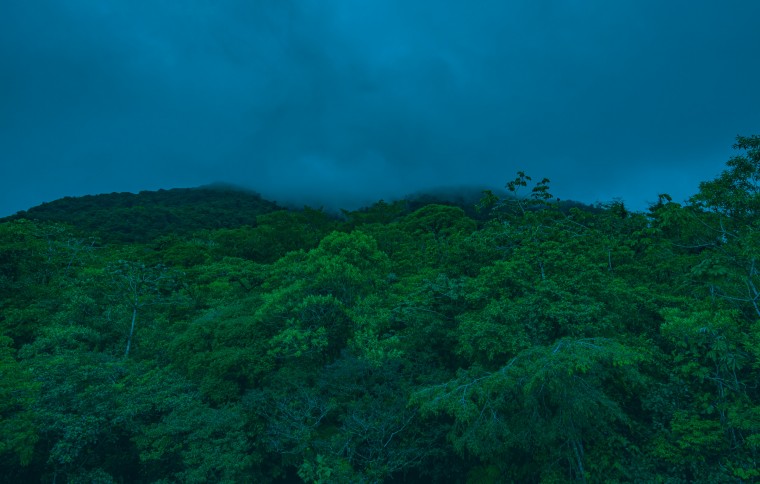This image captures a densely forested hillside, with lush, green trees that appear more vibrant towards the bottom. In the center of the picture, a gentle hill rises, covered in verdant foliage that continues up to the right-center where a notably taller tree extends beyond the right border. The scene is shrouded in low-hanging clouds or possibly fog, indicating a thick, misty atmosphere reminiscent of a rainforest. The sky, a dark blue suggesting an impending storm or the twilight hour, contrasts with the varying shades of green below. The top third of the photograph is dominated by the dense cloud cover, giving way to the rich, green vegetation that fills the bottom two-thirds, creating a moody, almost surreal landscape.